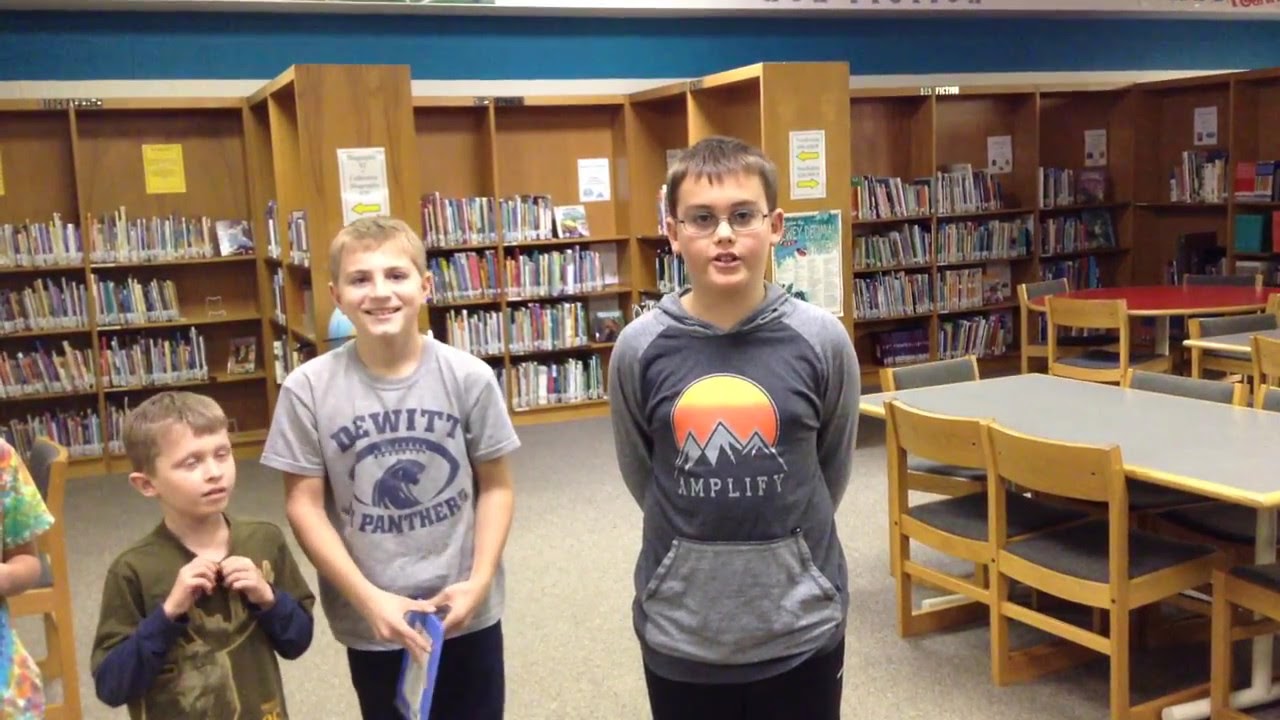The image depicts an elementary or middle school library, characterized by bookcases lining the entire back wall and a few extending perpendicularly into the room. In the right-hand side of the scene, there are tables: a round red one in the back corner and a light gray rectangular table in the foreground, both surrounded by wooden chairs. 

In the foreground on the left, three boys are standing and facing the camera. The boy in the center has short brown hair, wears glasses, and dons a dark gray and light gray hoodie with a mountain and sun illustration labeled "Amplify." He stands with his hands behind his back, mouth open, revealing his two front teeth. To his left is a boy with a short blondish hair, wearing a light gray t-shirt that features a football and the text "DeWitt Panthers." This boy is holding a book with his hands in front of him and is smiling. Next to him stands a shorter boy with short brown hair dressed in a greenish shirt over a long-sleeve blue shirt, looking slightly to the right. The left arm of another person, wearing a tie-dye patterned shirt, is visible at the leftmost edge of the image. 

Above the bookcases, a blue wall runs along the top of the image, and posters dot the ends of the shelves, enhancing the inviting atmosphere of the library.